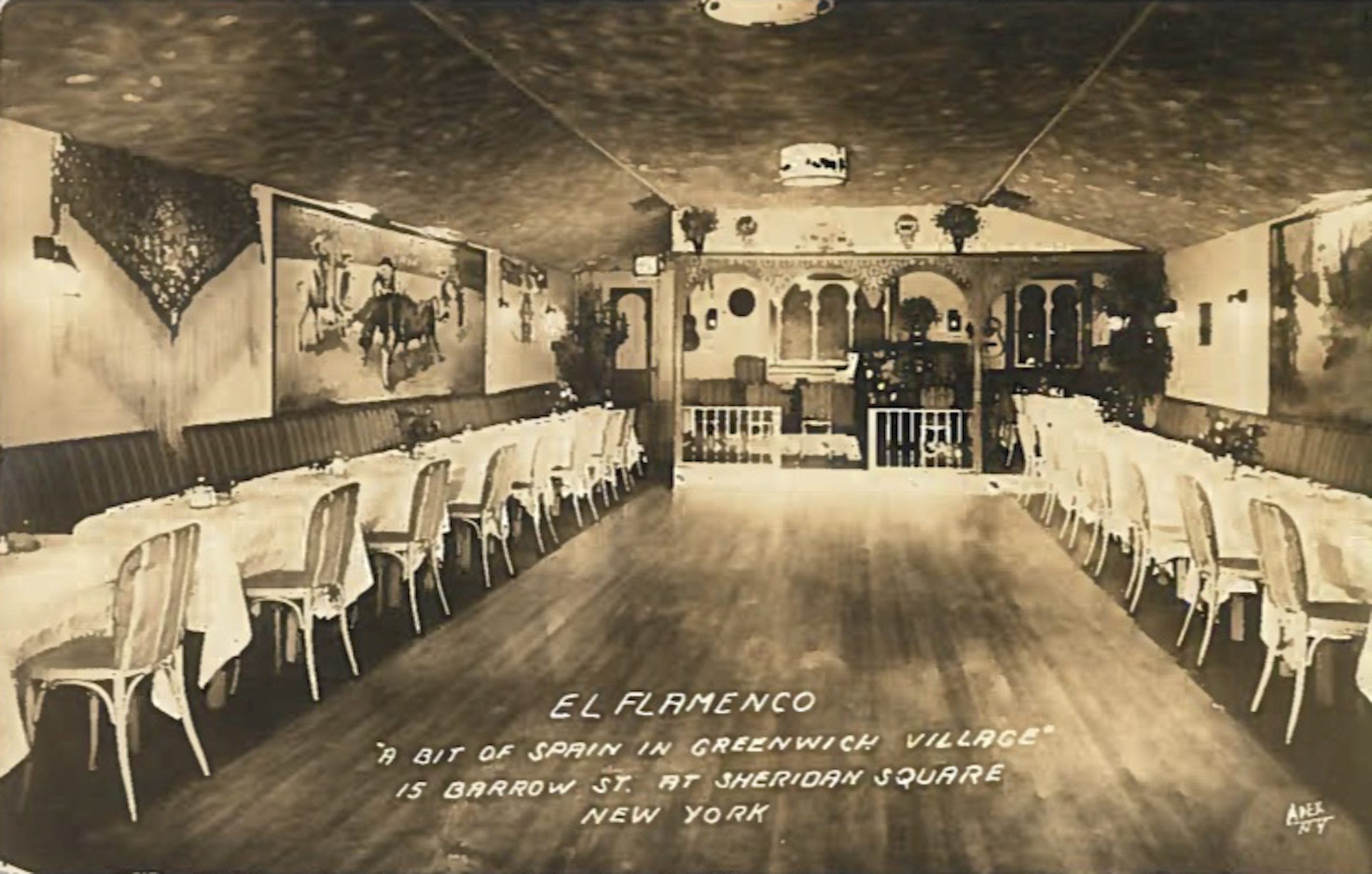This sepia-toned, black-and-white photograph depicts an elegant banquet hall or restaurant called "El Flamenco." The long, rectangular space features banquet-style booths along both sides, interspersed with evenly spaced tables. On the inner side, adjacent to the wooden floor that runs down the center, are rows of chairs, suggesting a layout designed for both dining and dancing. The ceiling is distinctively angled, resembling a gentler, triple-sloped roof. In the background, several archways lead to another seating area. The walls are adorned with various decorations and framed pictures, adding to the ambiance. Handwritten in white text at the bottom of the photo are the details: "El Flamenco, a bit of Spain in Greenwich Village, 15 Barrow Street at Sheridan Square, New York," with some initials and "NY" on the right side.